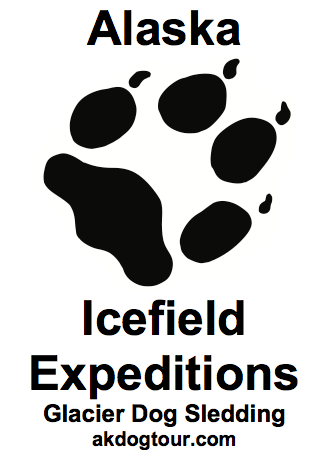The image features a minimalist design on a white background with black text. At the top, in a simple Arial font, it reads "Alaska." Below this is a large black paw print, tilted about 30 degrees to the right, showcasing four toes with visible small claws. Underneath the paw print, the text "Icefield Expeditions" is displayed, followed by "Glacier Dog Sledding" in smaller text, and finally "akdogtour.com" in even smaller text. The paw print, likely from a dog, is characterized by a rounded, misshapen oval shape at the bottom and more regular ovals for the toes, with teardrop shapes representing the claws. The edges of the text and image are slightly blurry, suggesting anti-aliasing effects. This image resembles a small black-and-white flyer or magazine ad promoting dog sled tours in Alaska.